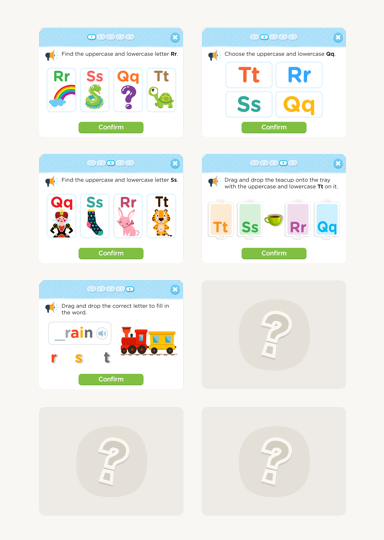This digital image features a collection of educational cards designed for children, each showcasing different letters of the alphabet along with corresponding images. The primary focus is on identifying uppercase and lowercase letters.

1. One card depicts a vibrant rainbow and includes both uppercase and lowercase 'R'.
2. Another card features a snake and displays uppercase and lowercase 'S'.
3. A card showcasing a question mark is paired with uppercase and lowercase 'Q'.
4. An endearing turtle is the centerpiece of a card that includes uppercase and lowercase 'T'.
5. Additionally, there's a card with an illustration of a queen, highlighting uppercase and lowercase 'Q'.
6. A colorful sock, decorated in black, yellow, pink, and blue, is the subject of another card, which includes uppercase and lowercase 'S'.
7. The image also contains a card with a pink rabbit, accompanied by uppercase and lowercase 'R'.
8. Finally, an animated tiger, colored orange and black, features on a card with uppercase and lowercase 'T'.

These cards form a visually engaging and educational tool for children to learn letter recognition through appealing imagery and vibrant colors.